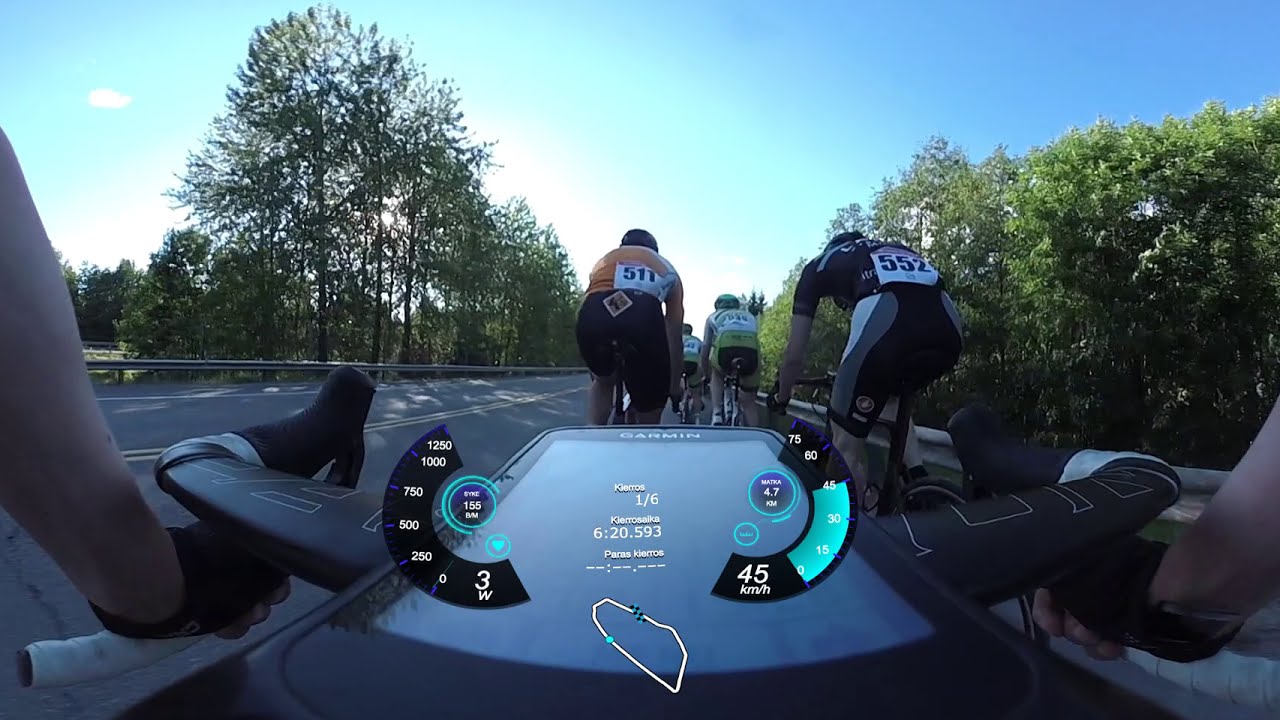In the image, captured from a first-person GoPro perspective, a bicyclist is racing down an asphalt highway through a rural area. The center of the photo features the cyclist's arms wrapped in black gloves gripping the downward-pointing handlebars, with a Garmin brand tablet mounted between them. Displayed on the tablet is a white line map marked by a blue dot, indicating the cyclist's position, alongside figures showing speed and total kilometers.

Ahead of the primary cyclist, several competitors ride toward the horizon, distinguishable by the numbers on their race tags and their attire. Prominently in the center-right of the image, a cyclist wearing a black shirt and black, gray, and white striped shorts, labeled with the number 552 on a white tag, pedals forward. Other cyclists sport orange, black, and yellow shirts. The road is bordered with green, leafy trees, and the serene scene is enhanced by a hazy bluish sky scattered with a few clouds. There is a clear double yellow line marking the center of the roadway, with all racers positioned to the right of it.